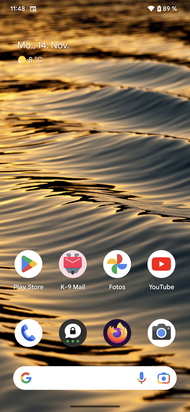The image depicts a device screen, possibly a smartphone or tablet. The top left corner displays the time as 11:48, while the top right corner shows Wi-Fi signal bars and a battery indicator at 89%, both in white. Below that, on the left side, it reads "Mo 14 November" and "8 degrees Celsius" with a sunny icon. The background features an image of water with reflective, gold and dark blue hues, showcasing ridges and movement without any frothing.

The screen includes several app icons: Play Store, K-9 Mail, Photos by Google, YouTube, and Phone. There's a text bubble with the phrase "let lock" and three green dots below it, potentially indicating a message notification. Additional icons include Firefox and a Camera. Below these is a Google search bar with the iconic "G" on the left and a microphone icon and photo icon on the right, in the recognizable red, blue, green, and yellow colors.